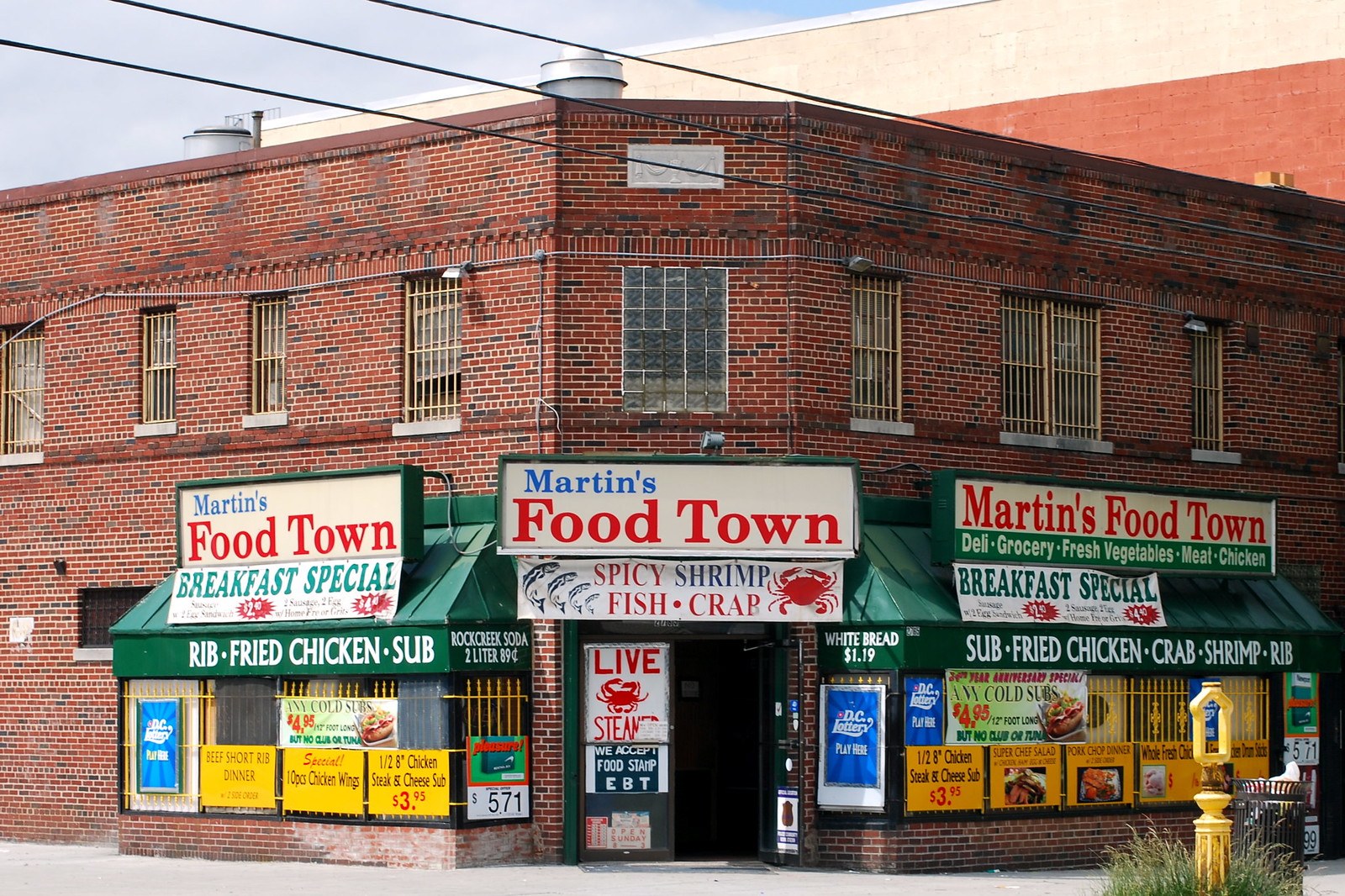The image depicts a two-story, red brick corner store named "Martin's Food Town" located under a partly cloudy sky. The store is situated at the intersection of two streets, with its main entrance angled and facing the corner. The larger building behind it features a combination of red and white bricks, while another cinder block building with a cream top and burnt orange bottom stands nearby. 

"Martin's Food Town" is prominently displayed in blue and red font on various signs around the storefront. Above the entryway, a sign advertises “Spicy Shrimp, Fish, Crab,” though the ‘B’ in "Crab" is partially missing. Additionally, the store has green awnings on either side of the entrance, displaying white text that reads "Sub Fried Chicken," "Crab," "Shrimp," and "Rib."

The scene includes numerous other signs indicating offerings such as "Live Steamed" with a crab illustration, "Breakfast Special," and a cigarette price of $5.71. The store also accepts EBT for food stamps, as indicated on one of the doors. Yellow security bars cover all windows, which run alongside both streets that form the corner. Power lines are visible in the foreground against the backdrop of a blue sky. The corner store is surrounded by various advertisements and informational signage, indicative of a bustling, urban bodega-like setting, possibly in Washington, D.C. There is also a D.C. lottery poster displayed, adding to the local character of the scene.